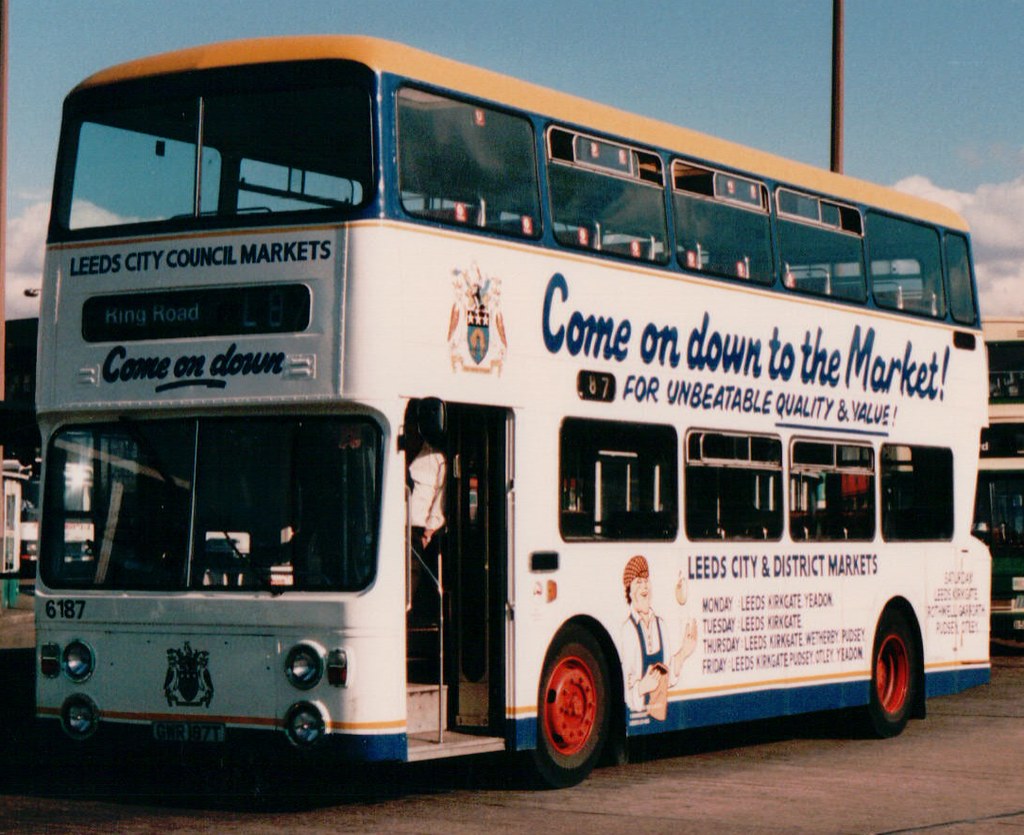This photograph captures a distinctive double-decker bus parked in a lot, serving as a promotional vehicle for Leeds City and District Markets. The bus is predominantly white with notable features: a tan or butterscotch-colored roof, a blue stripe along its bottom, and vibrant red wheels. A blue stripe also encircles the area around the windows. Emblazoned on its side, a slogan in blue lettering invites passersby to "come on down to the market for unbeatable quality and value." Below this, it lists several local markets and their schedules: "Monday Leeds, Kirkgate, Yeaton; Tuesday Leeds, Kirkgate; Thursday Leeds, Kirkgate, Weatherby, Posey; Friday Leeds, Kirkgate, Posey, Gottlieb, Yeaton." A charming cartoon image, presumably of a baker, adorns the side, reinforcing the market advertisement. The bus's front features a license plate and its door, located on the left side, is open, revealing someone standing on the top step. The overall color scheme of the bus mixes white, blue, and gold, creating a striking and easily noticeable vehicle that effectively promotes local markets.